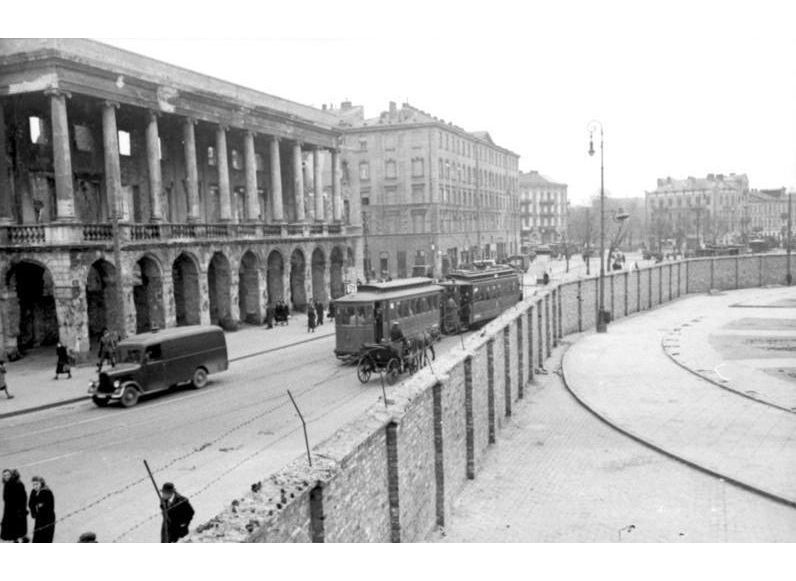The image is a highly intricate black and white photograph taken outside during the daytime. The scene depicts a bustling city street lined with old-style buildings featuring archways and columns on the left-hand side. The street is populated with a variety of vehicles, including a horse and buggy positioned towards the bottom center, and a two-car trolley pulling people further up in the middle of the picture. 

Numerous pedestrians, dressed in dark or black clothing, are seen walking along the street on the left. On the right-hand side of the image, a formidable wall runs from the lower left corner, curves around, and extends to the upper right corner. This wall is topped with barbed wire angled outwards, presumably to deter entry. Additional details include a significant light pole situated on the far side of this wall, and train tracks visible in the scene.

The atmosphere appears cold, possibly indicated by a white sky and what looks like snow on the ground. This image conveys a somewhat stark and perhaps tense urban environment, with architectural details and the presence of barbed wire hinting at a controlled or restricted area, adding to its historical significance.